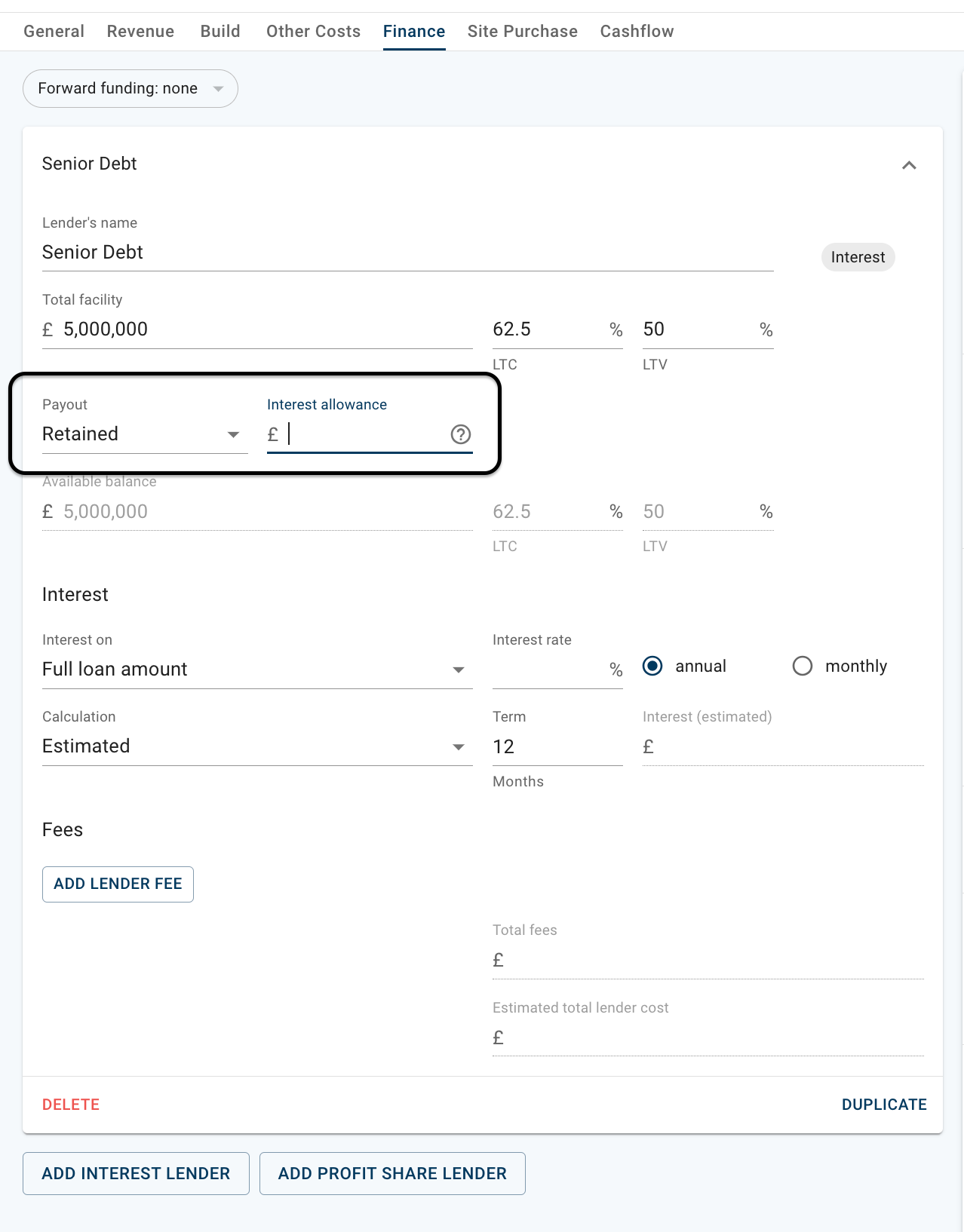The image showcases a detailed financial dashboard with various categories laid out horizontally across the top left section. The categories include General, Revenue, Build, Other Costs, Finance, Site Purchase, and Cash Flow, all written in a light grayish color except for 'Finance,' which is highlighted in blue and underlined. 

Beneath these categories, a bubbled bracket contains the label "Forward Funding: None." Below this, within a white rectangular area, the term 'Senior Debt' is prominently displayed at the top left. Descending downwards from this area, we find the label 'Leader's Name' followed by 'Senior Debt.' Further down, the term 'Total Facility' is listed with an underlying amount of $5,000,000. To the right of this figure, percentages are displayed: 62.5% and 50%, denoted further down by the abbreviations LTC and LTV, respectively.

Continuing below the $5,000,000 figure, the word 'Payout' and its subset 'Retained' are shown, alongside an 'Interest Allowance' section, which is currently blank. At the bottom left, the image features two bracketed areas: one labeled 'Add Interest Lender' and the other 'Add Profit Share Lender.'